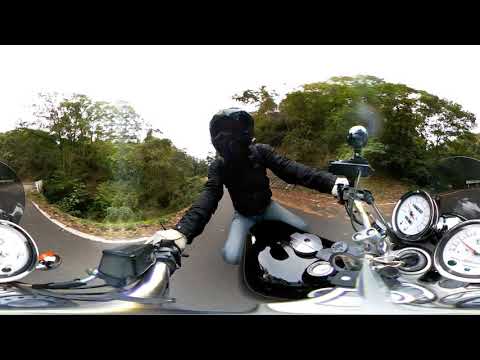A wide-angle photograph captures a motorcyclist riding down a single-lane, light gray asphalt road. The emphatic fisheye perspective causes a slight curvature in the scene. The rider is adorned in a black, full-face helmet with a shaded visor, obscuring their face, along with a black leather jacket, blue jeans, and white gloves. The handlebars of the black motorcycle are silver and feature multiple speedometers and gauges, though their readings are not discernible. The gray sky overhead, free of any visible clouds, casts a stark, muted light on the surroundings. On both sides of the road, vibrant green-leaved trees mark the landscape. The road itself is bordered by a small white curb, adding a touch of structure to the otherwise fluid scenery. Smoke trails faintly from the motorcycle, adding a dynamic sense of motion as the biker cruises through the daytime outdoors.